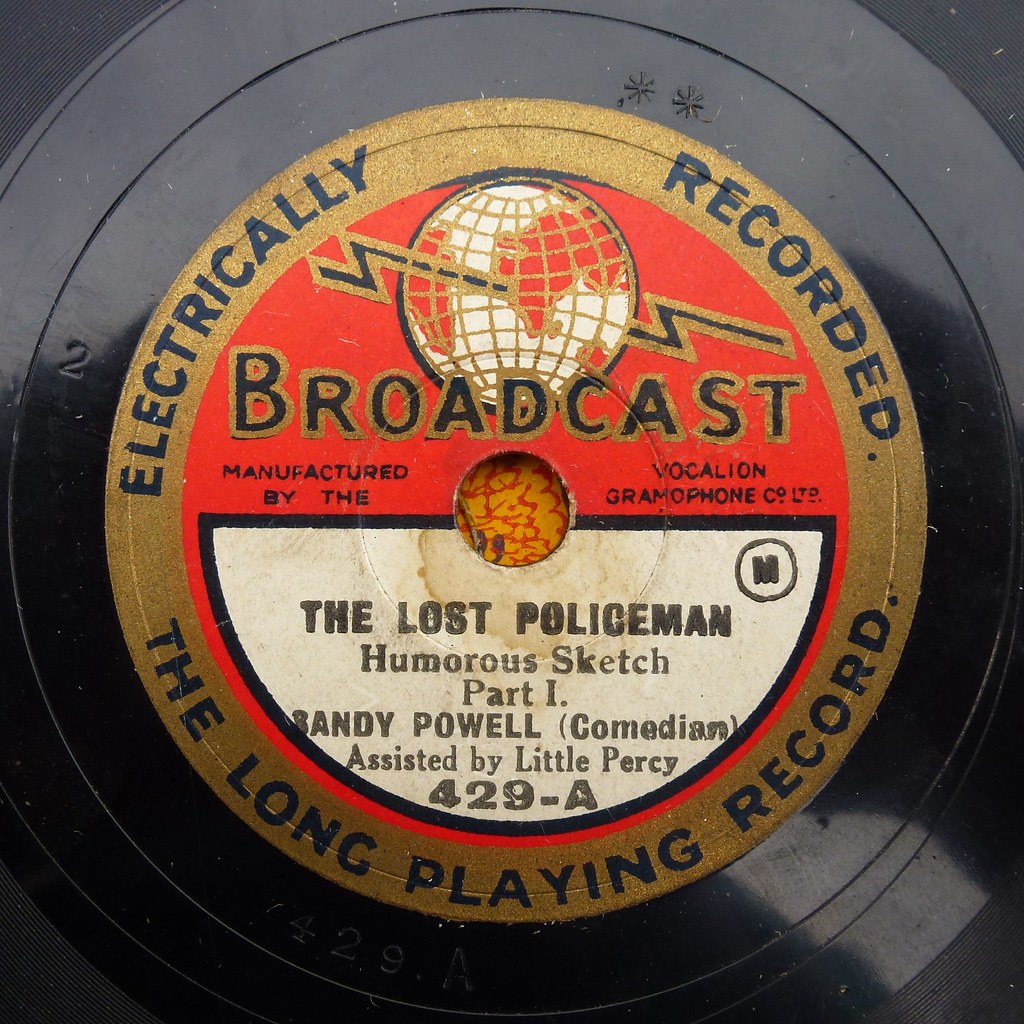The photograph captures a close-up of a vinyl LP record, prominently showcasing its central label. The outer edge of the record is shiny and black, with visible grooves. The label itself is intricately designed with a gold border encircling a vivid red center, and features a distinctive white semi-circle at the bottom of the red section. The gold border contains the black text: "Electrically Recorded The Long Playing Record." Within the red center, it reads: "Broadcast, Manufactured by The Vocalion Gramophone Company Limited." The white semi-circle at the bottom of the red section lists the details: "The Lost Policeman, Humorous Sketch Part 1, Randy Powell Comedian, Assisted by Little Percy." Additionally, the catalog number "429-A" is inscribed. Within the red portion of the label, there is an image depicting the Earth with a lightning bolt emerging from either side, adding a unique visual element to the design.